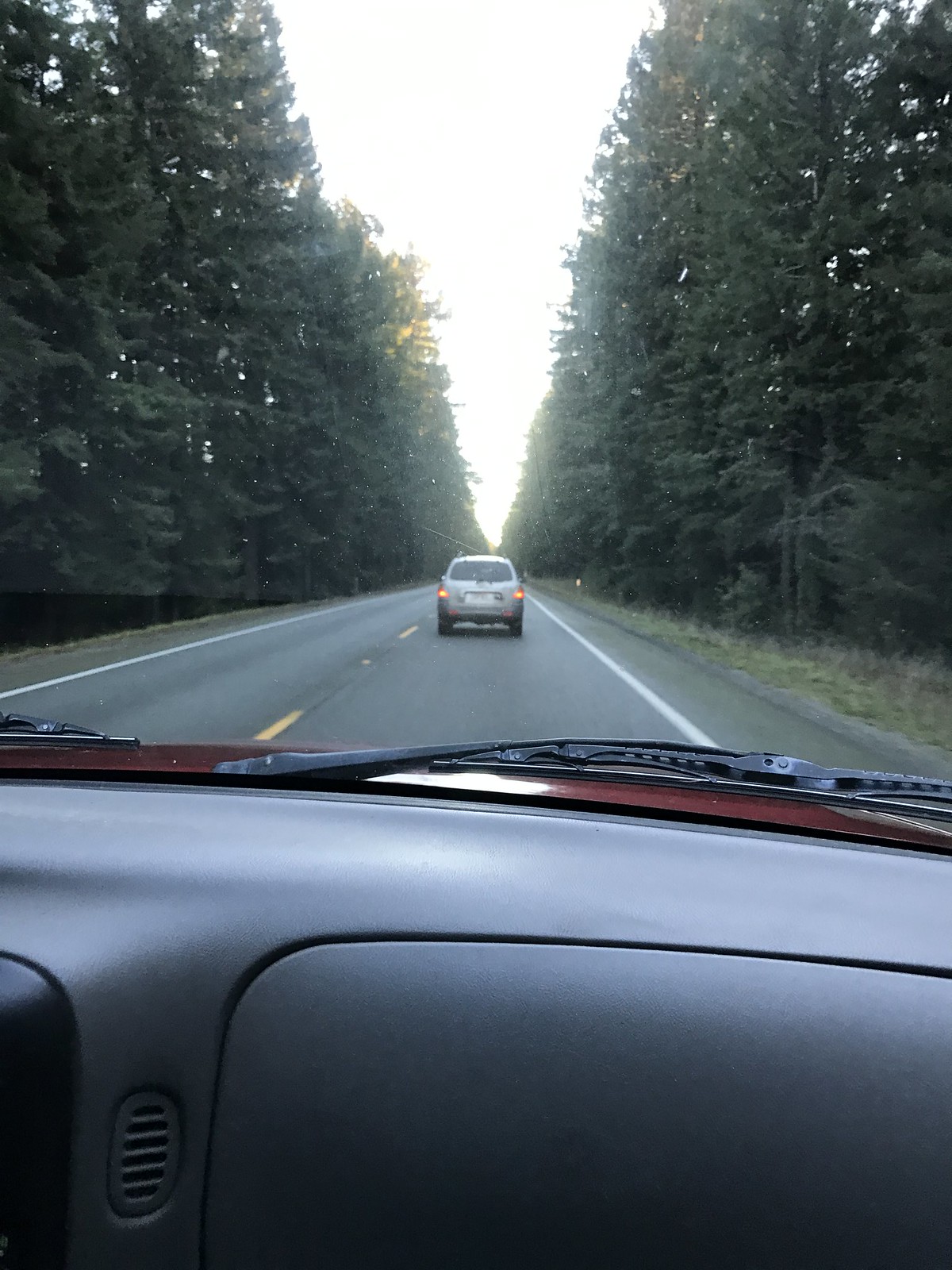A daytime photograph captured from the perspective of a seated passenger inside a vehicle shows a view through the slightly dirty windshield. The dashboard is partially visible at the bottom edge of the image. The vehicle is traveling down a well-maintained concrete road, distinguished by white lines on the sides and a yellow line dividing the center. The scene is set in a heavily wooded area with dense green foliage and towering trees flanking both sides of the roadway. Directly ahead, a gold-colored van drives along the same path. Rays of sunlight peek through the tree canopy above, casting a gentle glow over the scene. Patches of green grass of varying heights can be observed along the road's edge, contributing to the lush, verdant atmosphere.